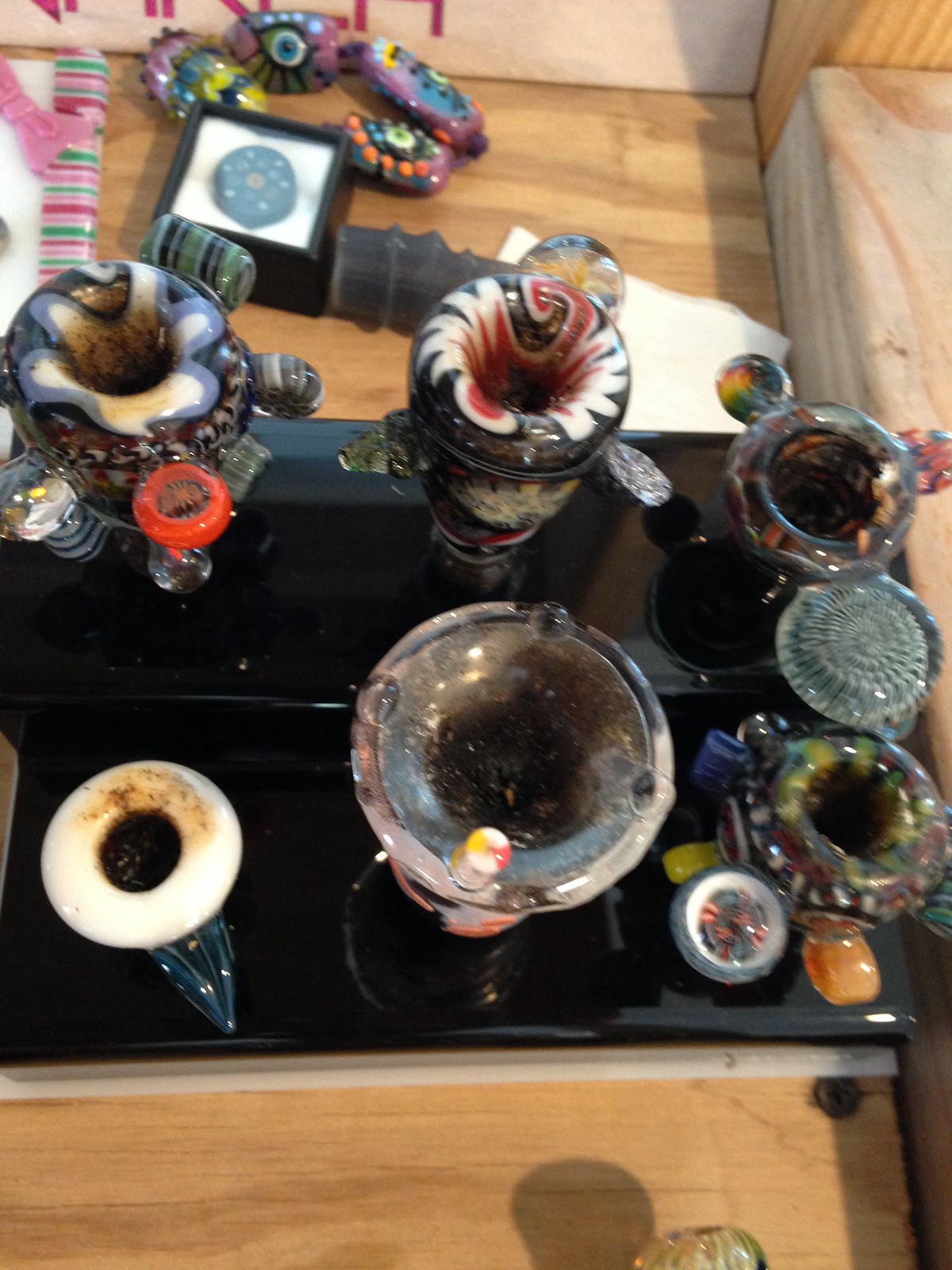The image depicts an eclectic collection of intricate, colorful glass and ceramic objects, predominantly resembling hookahs, bongs, or artistic smoking devices. These vessels showcase a wide array of shapes and designs, including donut-like forms, swirling patterns, and handles. Many of them feature psychedelic, rainbow hues and some even have eye motifs or floral decorations.

The objects are arranged atop a shiny black tray, which rests on a wooden surface with visible grain, possibly resembling a table or a step. The composition appears slightly out of focus, adding to the mystique of the scene. In the background, there are additional glass or ceramic items, including some that look like painted stones with vibrant colors such as purple, blue, orange, and light green.

The overall setting gives the impression of a whimsical, almost surreal display of both used and pristine objects, blending functionality with artistry. A shadow and a pink and green striped item are visible on the wooden surface in the bottom corner, contributing to the detailed, multifaceted environment captured in the photograph.